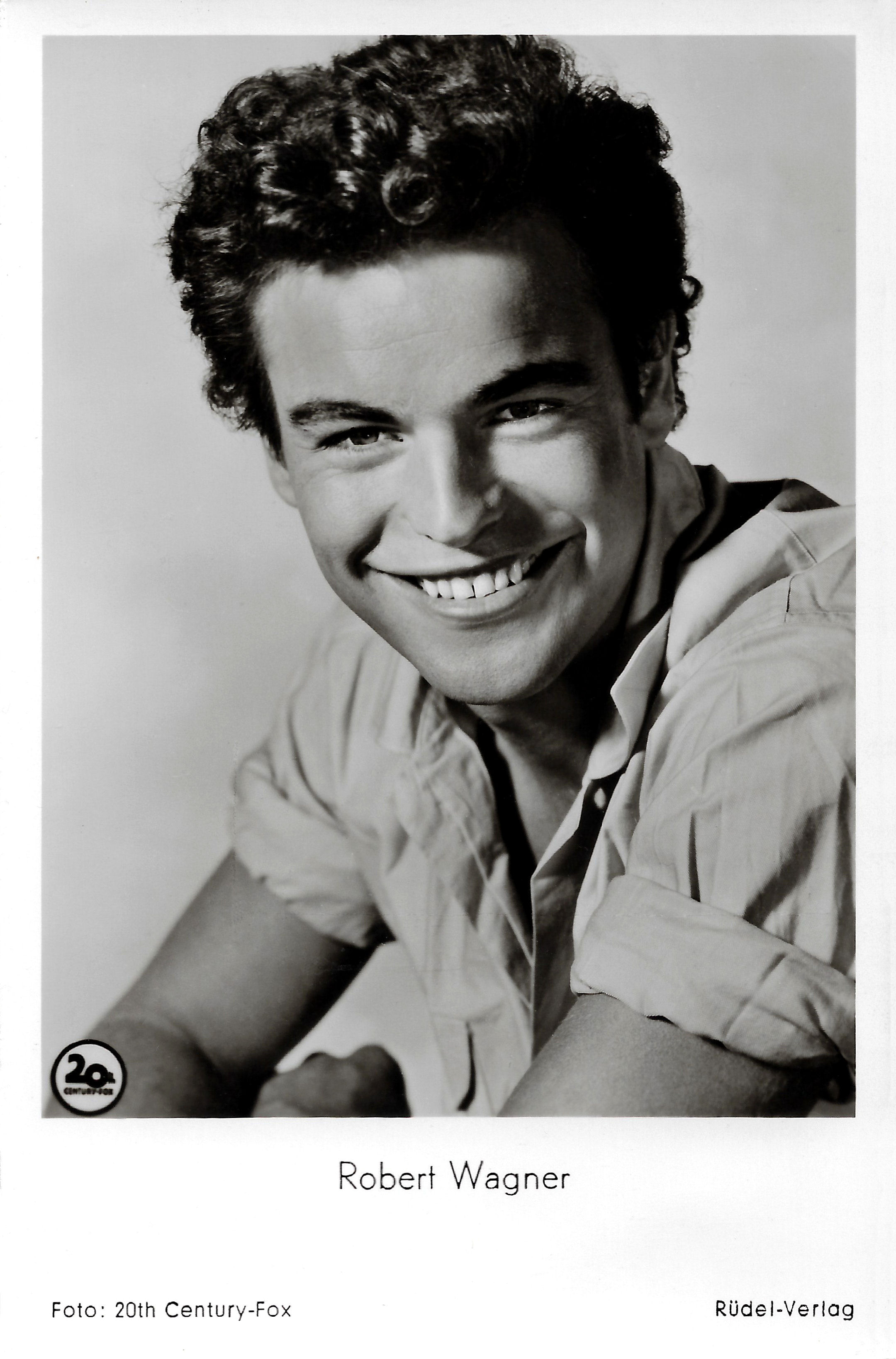This photograph is an older headshot of the renowned actor Robert Wagner, likely taken around 20 years ago when he was in his late 20s. Wagner is depicted with shorter, curly hair that frames his face. He is smiling, revealing his teeth with his lips slightly parted. The actor is dressed in a long-sleeve, white button-up shirt with the sleeves rolled up to his biceps. His arms are crossed as he looks directly into the camera, exuding a confident yet approachable demeanor. The bottom left corner of the image features an older version of the 20th Century Fox logo, while the words "Robert Wagner" appear beneath his picture in a smaller black font. Below his name, in an even finer print, the caption reads "Photo 20th Century Fox" on the left side and "Rudel Verlag" on the right side.